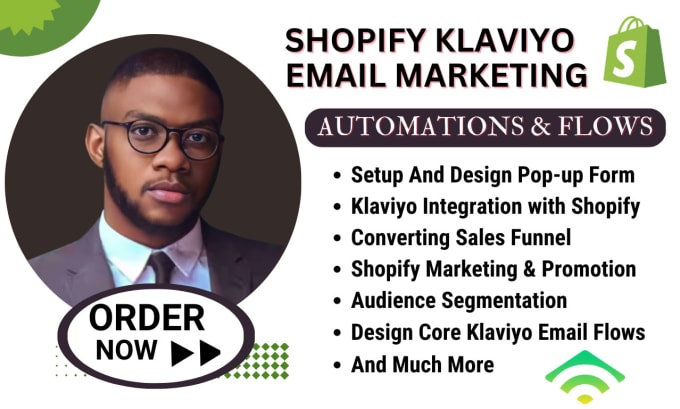This horizontally rectangular advertisement presents a clean white background with several key elements and text, focusing on promoting Shopify's Klaviyo email marketing services. 

In the upper left corner, a green arc transitions into a lighter green shade off the image's edge. Below and slightly to the right, a circular inset features a close-up of a man with short, dark hair and a lightly bearded face. He wears round black glasses, a gray suit jacket, a white collared shirt, and a dark tie against a brown background.

Adjacent to this, an elongated black bubble contains "automations and flows" written in white letters. Underneath, seven bullet points in black detail the features: setup and design pop-up form, Klaviyo integration with Shopify, converting sales funnel, Shopify marketing and promotion, audience segmentation, design core, Klaviyo email flows, and much more.

The central part of the ad prominently displays "Shopify Klaviyo email marketing" in bold black letters, accompanied by the Shopify logo—a green shopping bag with a white 'S'. To the left, a button outlined in black reads "order now" with two black arrows pointing right, and it is accentuated by green dots.

Finally, in the bottom right corner, an emblem in green, white, and yellow adds a final touch to the comprehensive layout.